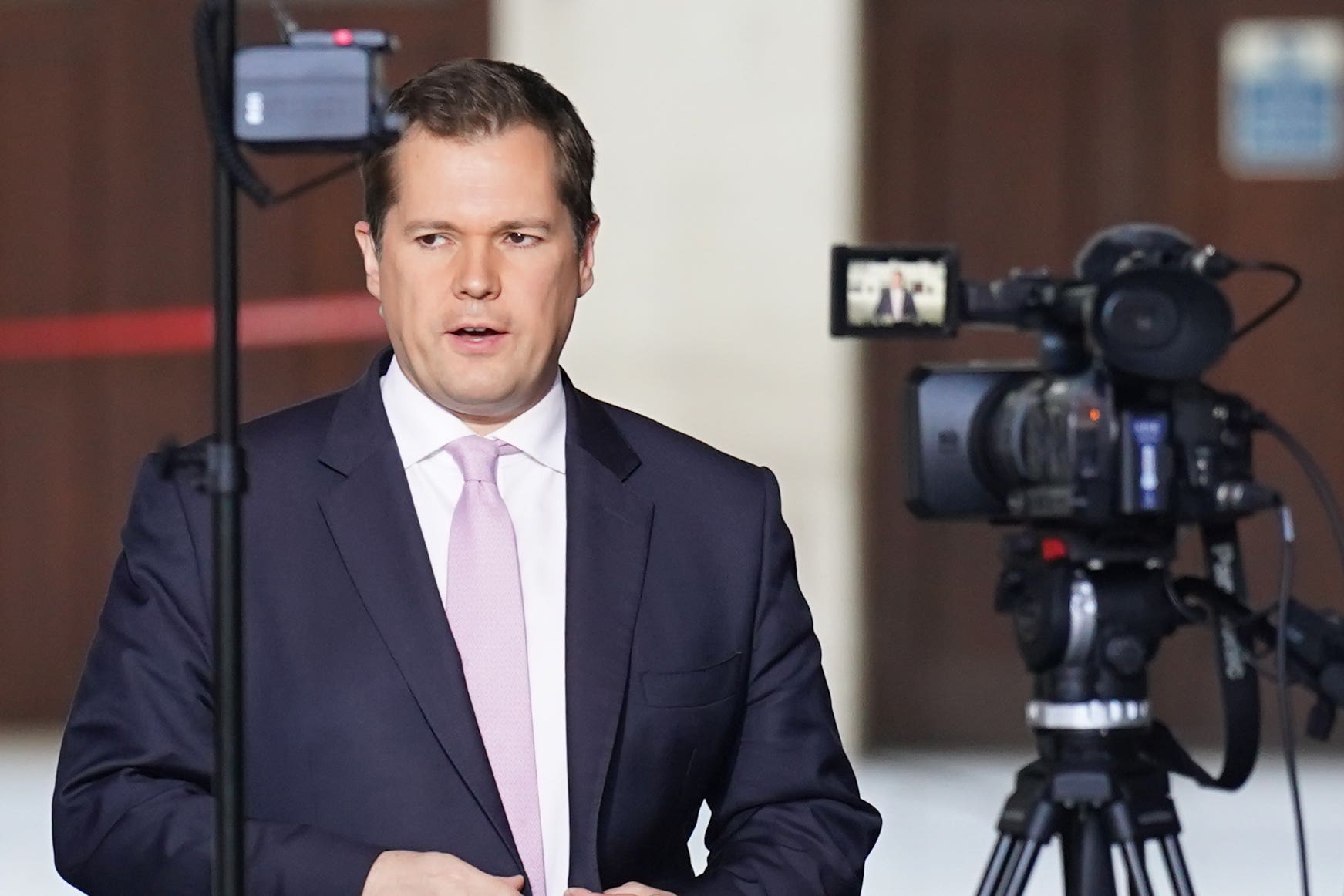This photograph features a clean-cut Caucasian man with short dark brown hair, wearing a dark blue suit, a white dress shirt, and a dusty rose-colored tie. He stands from the elbows up with a serious expression, his mouth slightly open as if speaking, and his hands mid-motion, possibly buttoning his suit. Positioned in front of him is a sleek black camera on a tripod, its small LED screen displaying his image. The scene appears to be set up for a recording, perhaps an interview or news segment. The background comprises a dark brown wall with a broad vertical white stripe running through the middle, lending to the impression of a studio environment. Additionally, there's a potential light or light sensor mounted to the left, suggesting professional lighting. The cables and equipment associated with the camera are also predominantly black, maintaining a uniform aesthetic in the setup.